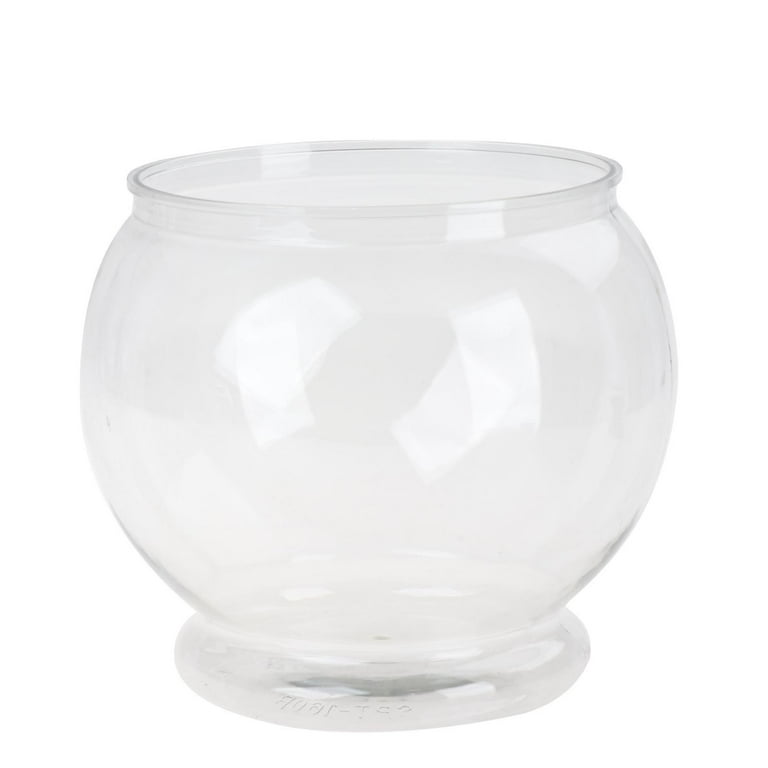The image depicts a plain, transparent glass fishbowl centered against a stark white background. The fishbowl is predominantly spherical with a circular opening at the top and a rounded pedestal base at the bottom. It appears empty, with no water or fish inside, highlighting its simplicity. A faint etching of letters and numbers is barely visible on the bottom center of the bowl, adding slight detail to its otherwise clear surface. Light reflections can be seen at the top and center of the bowl, contributing to its see-through appearance. The entirety of the scene emphasizes the glass texture and minimalistic design, devoid of any additional colors or text, set in an indeterminate white space.